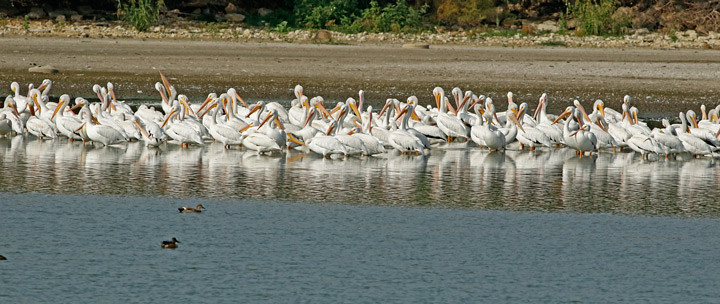The photograph portrays a vibrant coastal scene from a boat, taken from a short distance out to sea, offering a detailed view of the shoreline. The water is divided into two distinct bands of color: nearer to the viewer, it displays a murky bluish-green hue, home to a pair of ducks—a mallard and a female—calmly bobbing on the surface. Further in, the water transitions to a crystal-clear state, where the stony pebbles of the shoreline are easily visible.

Dominating the shoreline is a striking assembly of at least 50 American white pelicans, their pristine white feathers and long orange beaks standing out against the backdrop. The pelicans form several rows stretching from the left to the right side of the image, with some depicted preening or grooming themselves and each other in a seemingly tranquil harmony. Their reflections shimmer in the water, creating a mirror-like effect, while a few of their legs are visible just above the waterline. To further enrich this picturesque scene, the tide is out, exposing additional rocky patches along the coast where the pelicans are interspersed, mingling at this juncture of land and sea, making for a compelling and dynamic landscape.